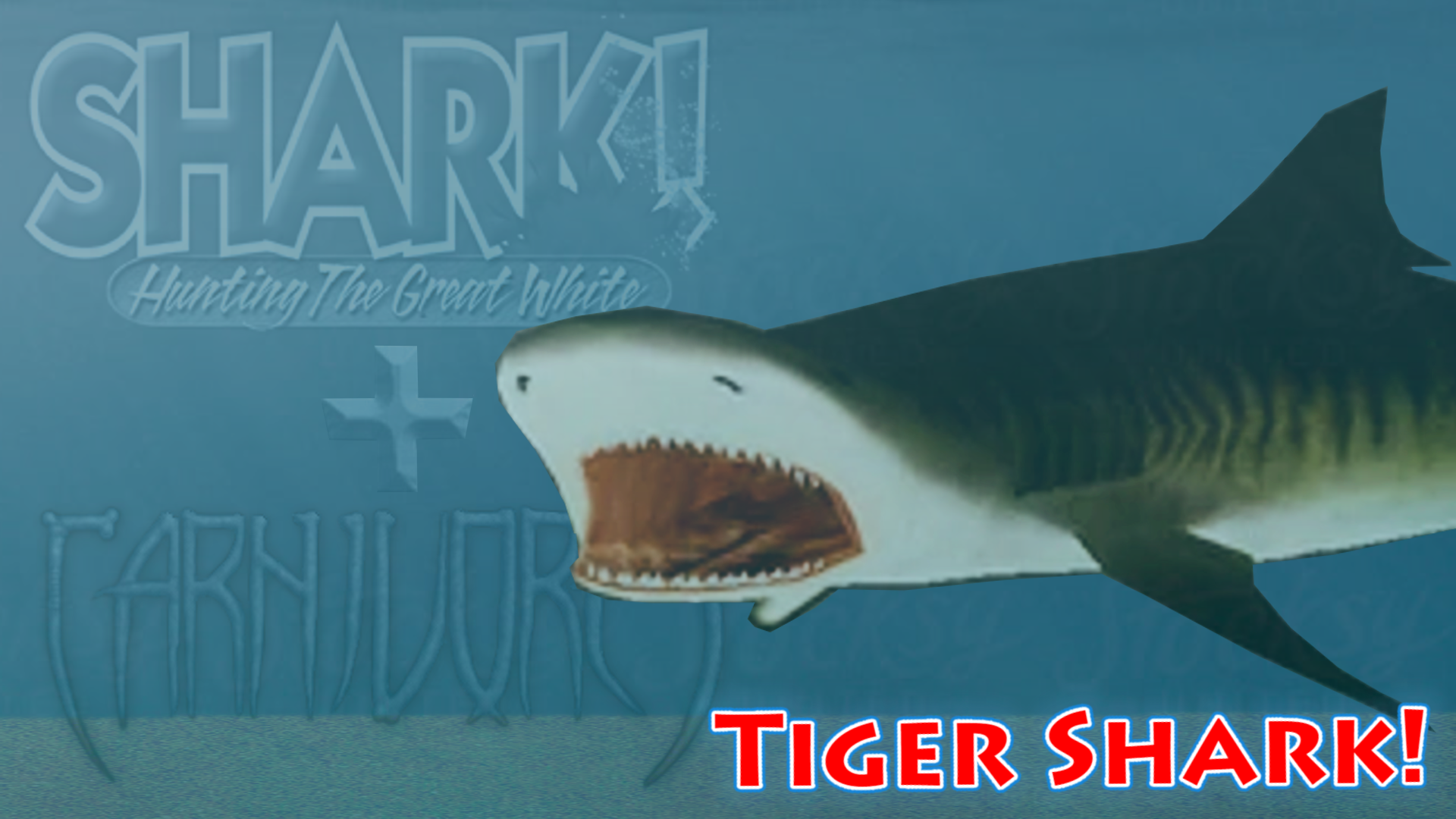The image appears to be a poster with a blue background that transitions to a lighter blue at the bottom, giving an underwater effect. On the left side, there's bold, light white text reading "SHARK!" followed by subtext in cursive that says "hunting the great white." Below this, a cross symbol is visible, and underneath it in parentheses, the text appears blurred or unclear. Dominating the right side of the image is an animated depiction of a shark, specifically a tiger shark, with its mouth wide open, showcasing sharp teeth and a red interior. The shark's bottom half is white while the top is gray with dark and light striations. The animal's nostrils are visible, but its eyes are not. In the lower right corner, bold red text framed in white outline declares "TIGER SHARK!" This detailed depiction likely serves an educational or illustrative purpose, possibly for an online article, children's book, or blog post about shark species and their behaviors.